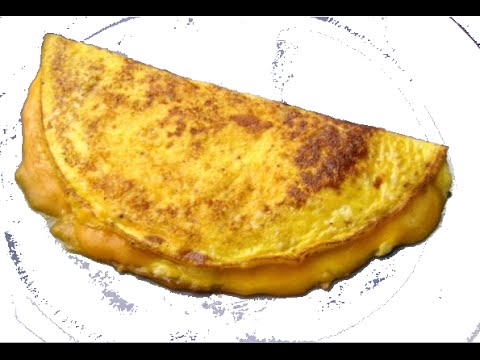The image depicts the outline of a white plate, rendered in a sketch-like, superimposed style with gray lines that resemble a simple illustration. On this plate sits a bright yellow omelette, perfectly folded into a half circle. The omelette has visible signs of melted cheddar cheese oozing out from its middle, giving it a gooey, appetizing appearance. There are slight burnt spots along its edges, with one corner appearing more charred than the rest. The top and bottom of the image feature thin black lines running across the page, framing the bright yellow omelette and enhancing the overall composition.